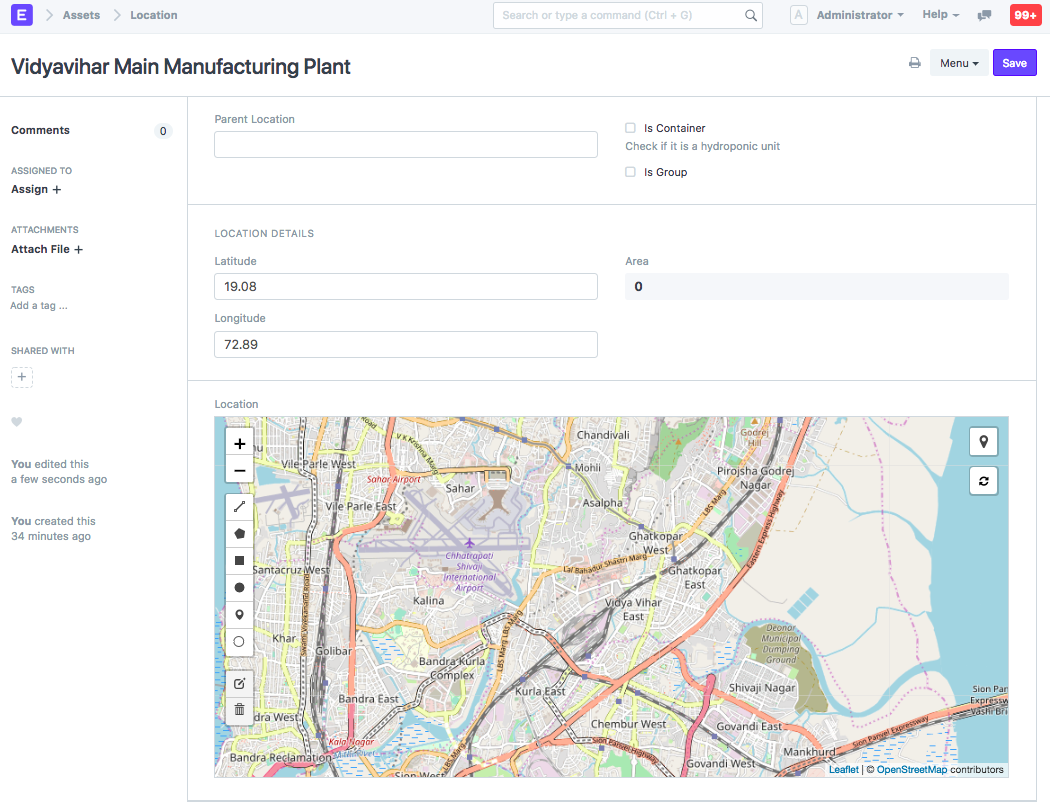Here is a cleaned-up and detailed caption for the described site image:

---

The website interface appears to pertain to a business application, featuring a variety of tools and navigation options. In the upper left corner, there is a prominent "E" logo. Directly below this, labels for "Assets" and "Location" are displayed. At the top center of the page, a search bar is provided for quick navigation, while the top right corner houses icons for the administrator panel and help resources.

Beneath the search bar, there's a red notification field displaying "99+" alerts, alongside a print option menu. To its left is a purple "Save" button. The main header section reads "Vidya Vihar Main Manufacturing Plant."

Along the left sidebar, the user can navigate through several options including "Comments," "Assign To," "Assign +," "Attachments," "Attach File +," "Tags," "Add a Tag," and "Share With +." Additionally, a heart icon indicates favorited items.

User activity is noted with prompts such as "You edited this a few seconds ago" and "You created this 34 minutes ago." Moving to the right of this information, there is an input field for "Parent Location" followed by several unchecked checkboxes labeled "Is a container," "Check if it's a hydroponic unit," and "Group." 

A detailed bar stretches across the width below these fields, segmenting the interface. In a secondary section above a map display are the "Location Details," including latitude (19.08) and longitude (72.89) coordinates, and an area labeled "0."

The map displayed below encompasses a street and city overview, resembling Google Maps but actually powered by Leaflet with OpenStreetMap contributors. The bottom of the map area features a subtle gray line.

---